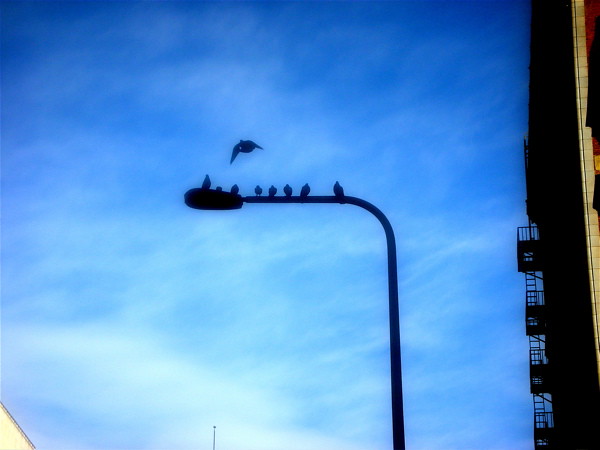The photograph captures a serene yet detailed scene, possibly at dusk, featuring a silhouetted streetlight prominently in the center. The lamp post extends upwards from the bottom of the image, curving slightly to the left, terminating in an oval-shaped lamp head. Perched atop the horizontal bar of the streetlight are nine birds, with one more in mid-flight, about to join them. Dominating the background is a gradient blue sky accented with light clouds, creating a tranquil atmosphere. On the right side of the image, an imposing silhouette of a building—likely a high-rise apartment—stretches from top to bottom, revealing four sets of fire escapes. The building's dark outline contrasts sharply against the sky's softer hues, enhancing the overall silhouette effect of the scene.